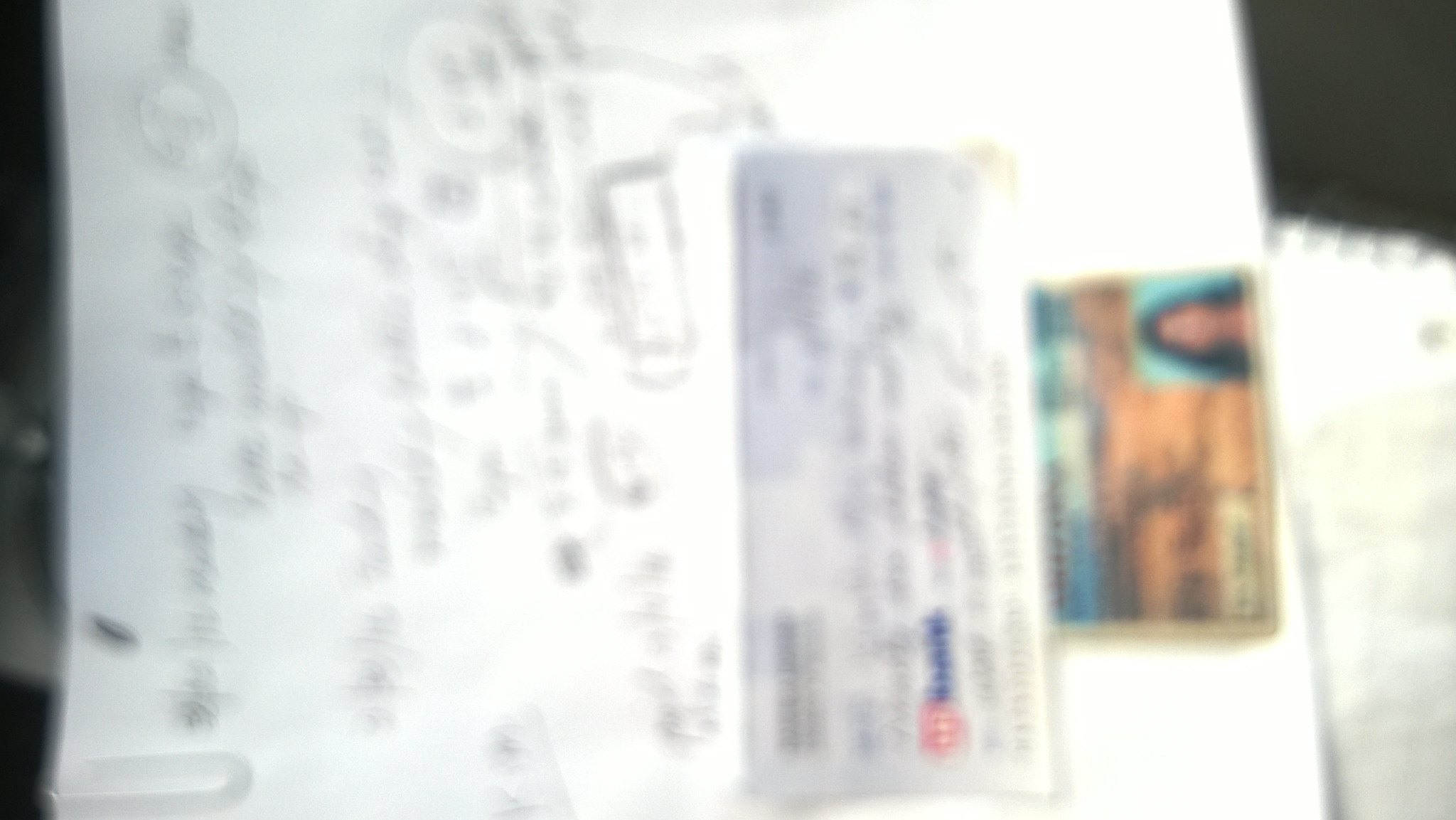The image depicts a severely blurred view of personal documents. In the foreground, a driver's license features a woman with long black hair, though specific details remain indistinguishable. Alongside the license, a check from U.S. Bank is visible, identified only by the recognizable logo. Behind these items lies a piece of paper with additional written information, fastened by a paperclip in the corner. The overall color scheme includes hues of black, white, red, blue, and brown, adding a mosaic of indistinct colors to the blurred imagery. The lack of clarity serves to protect the sensitive information presented.